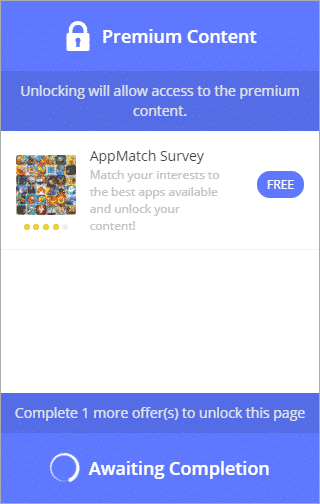The screen displays a user interface with a predominant purple and white color scheme. The top and bottom sections of the page are highlighted with a light purplish-blue gradient. At the very top, within a border, bold white text reads "Premium Content." Adjacent to this text is a white lock icon symbolizing restricted access to certain content.

Beneath this section, explanatory text indicates that "Unlocking will allow access to the premium content." The detailed message suggests that completing an "App Match Survey"—aligning user interests with the best available apps—will grant access to the locked content. 

This information is presented on a white background, accompanied by a vibrant thumbnail featuring colorful images. Next to the thumbnail is a prominent purple button labeled "Free" in white text.

At the bottom of the screen, a message prompts the user with: "Complete one more offer to unlock this page." To the right, a white circular loading icon is shown, along with the words "Awaiting completion" in a bold white font.